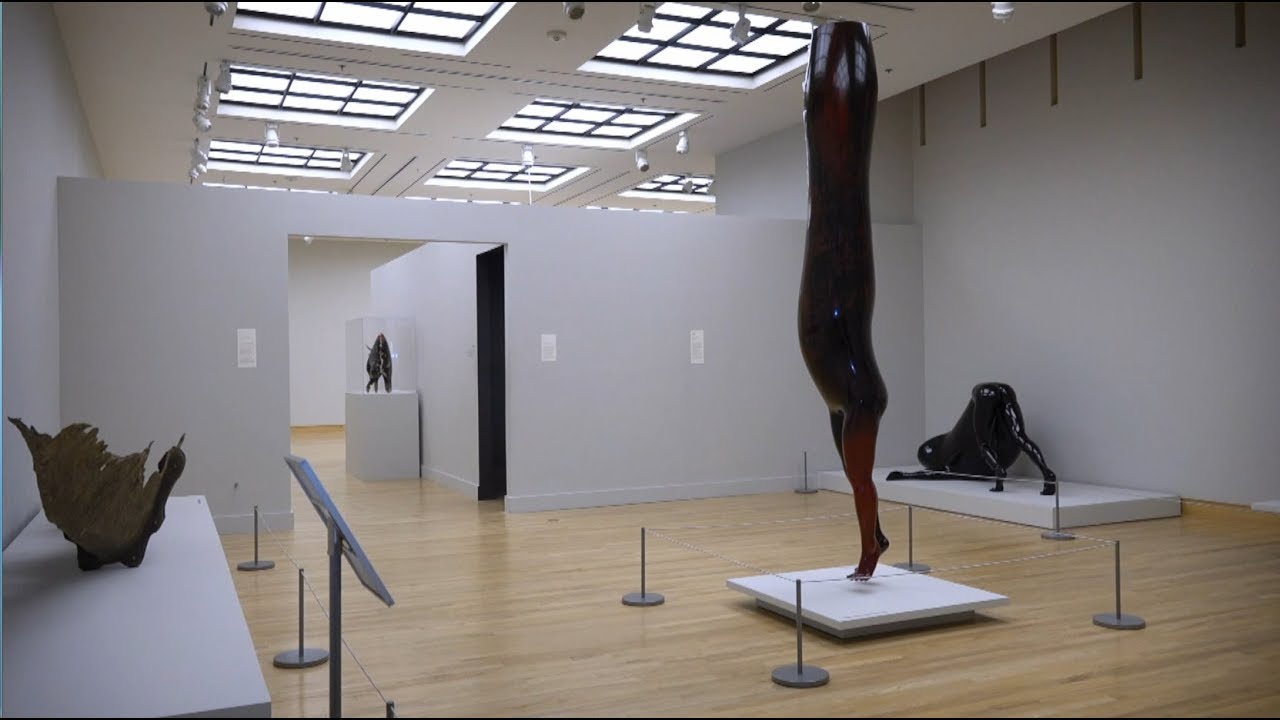The photograph depicts an art gallery with light brown hardwood floors and plain gray walls, contrasted by a white ceiling featuring sunroof panels and recessed lights. Dominating the space are four distinct sculptures on white platforms, each framed by rope barriers supported by four posts. The central piece commands attention: a substantial black figure resembling a human form with legs poised on tiptoes, extending seamlessly into a large, smooth black mass that nearly reaches the ceiling. Nearby, a similar black sculpture appears as if a body is bent over, legs forming an upside-down V against a white stand. To the left, there is a small table displaying another sculpture and near the doorway to another room stands a platform with a small, indistinct statue inside a glass case. In the background, there seems to be a part of an animal figure, possibly a cow, with sections missing, also placed on a white stand. Detailing includes a placard positioned next to the central piece and numerous ceiling lights illuminating the exhibits, adding a sense of depth and focus to the arrangement.